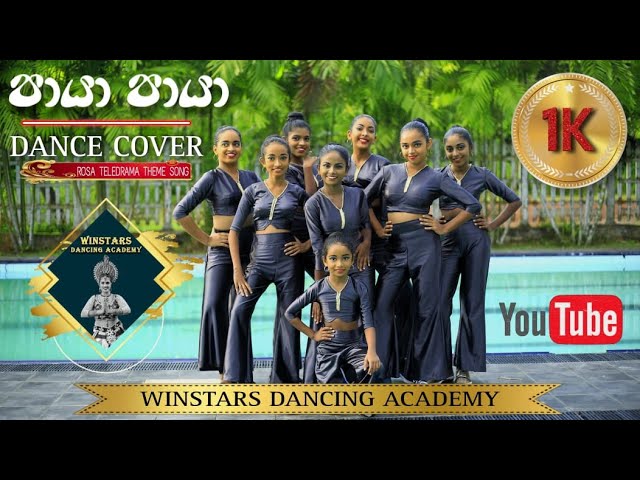This is an advertisement from YouTube promoting the WinStar Dancing Academy. The image features a group of young ladies, likely of Indian descent, given their dark skin and black hair. They are all smiling and showcasing their dance attire, which includes black crop tops with elbow-length sleeves, gold earrings, and black bell-bottom pants. Their hair is styled in buns. They stand against a green background near a pool and a fence, with lush greenery in the distance. The text in the image includes "dance cover" and some phrases in a non-English language. There is also a red rectangle with delicate white text reading "Rosa Teledrama Theme Song," and a gold circle with red letters denoting "1,000." At the bottom, a yellow ribbon advertises the WinStar Dancing Academy.